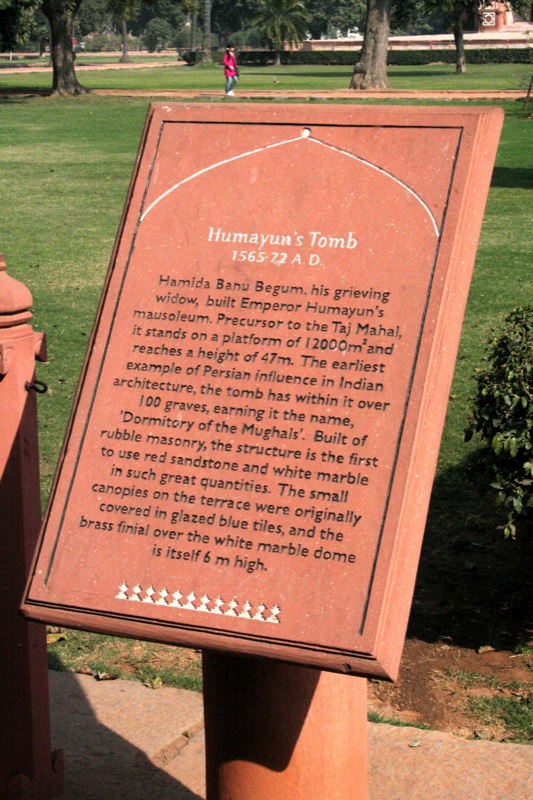The image captures an outdoor scene featuring a reddish-brown stone plaque mounted on a cylindrical stone pillar, slightly tilted in the photograph so the right upper and lower portions appear closer. The plaque is inscribed with detailed historical information in white and black text. It reads, "Humayun's Tomb, 1565-72 AD," and describes that Hamida Banu Begum, the grieving widow of Emperor Humayun, built the mausoleum. As a precursor to the Taj Mahal, the tomb stands on a 12,000 square meters platform and rises to a height of 47 meters. This site, the earliest example of Persian influence in Indian architecture, contains over 100 graves, earning it the title "Dormitory of the Mughals." Built using rubble masonry and notable for its extensive use of red sandstone and white marble, the tomb originally featured canopies covered in glazed blue tiles and a six-meter high brass finial atop the white marble dome. The background shows a sunny day in a green park with large tree trunks, a bush to the right of the plaque, and a person wearing a pink or bright red coat and white shoes walking on a brown stone path. A small stone structure is visible to the left of the plaque.